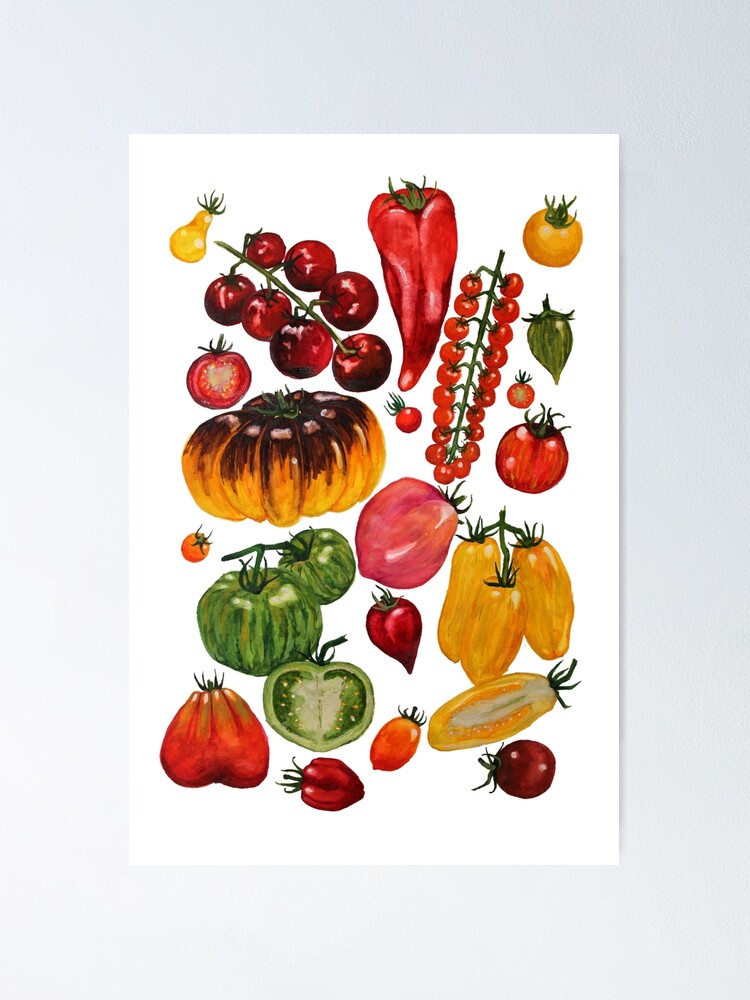This vibrant and detailed poster or book cover showcases an artistic depiction of various fruits and vegetables against a crisp white background. Dominated by shades of red, yellow, orange, and green, the painting features a mix of colored pencil drawings and potentially AI-generated prints. The composition includes strings of cherry tomatoes, red bell peppers, yellow long tomatoes (one of which is halved), and an heirloom tomato with a yellowish-purplish-brown hue. Scattered across the image are single cherry tomatoes and a mix of other small tomatoes. 

On the left side, there is a green-hued trio of vine tomatoes, and towards the bottom right, three yellow long tomatoes accentuate the scene. Among the vibrant produce, there is also a gourd, brown at the top and orange at the bottom, a small yellow pear, red cherries, and curvature-shaped yellow bell peppers. Each element is meticulously illustrated, emphasizing the diversity and vividness of these natural forms. The overall clean and crisp presentation reinforces the freshness and appeal of the depicted items, making for a captivating visual experience.